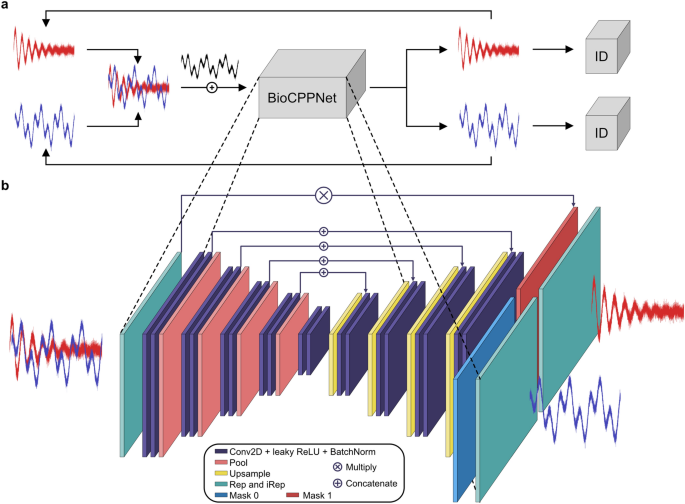This detailed diagram depicts the inner workings of a technical product. At the top, long horizontal arrows and wavy structures in red, blue, and black, resembling sound waves, converge towards a central silver or gray box labeled "biocpp.net." Dotted lines extend downward from this box to arrays of color-coded rectangular panels. These panels are depicted at an angle, showing many layers featuring colors such as blue, red, green, yellow, pink, teal, and purple, which shrink towards the center and expand again towards the right. At the bottom, a key explains the colors, indicating that blue represents mask 0, red represents mask 1, yellow stands for unsample, and other colors correspond to terms like CONV2D, LEAKY, RELU, POOL, UNSAMPLE, REF, and IREF. Flowcharts and additional wavy lines further illustrate the interaction between various components in the diagram. The diagram is segmented into two parts, labeled A and B, with arrows and electrical-like symbols connecting different sections, providing a comprehensive view of the processes involved.